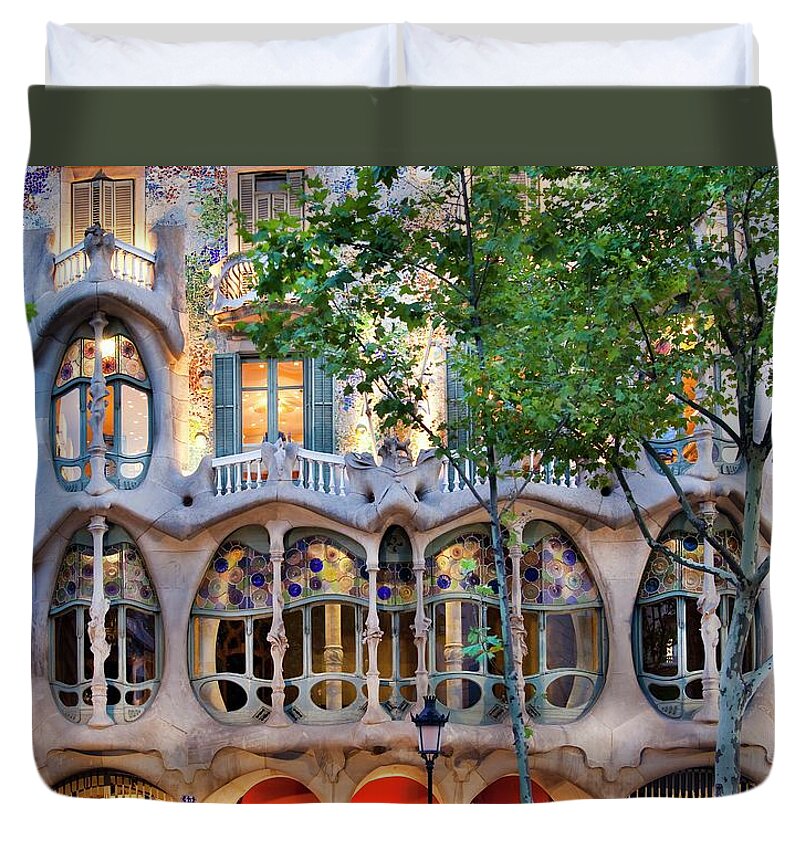The image showcases a quirky, multi-storied building with a wavy structure and numerous circular windows, some adorned with wooden shutters and glass panes. This gray building, standing tall with almost four visible levels, features balconies with white railings and stained windows in blue and yellow hues. Tall, lush green trees add a natural element outside the building, complementing the unique architecture. Captured in daylight, the setting evokes a sense of European charm, reminiscent of an amusement park's whimsical design.